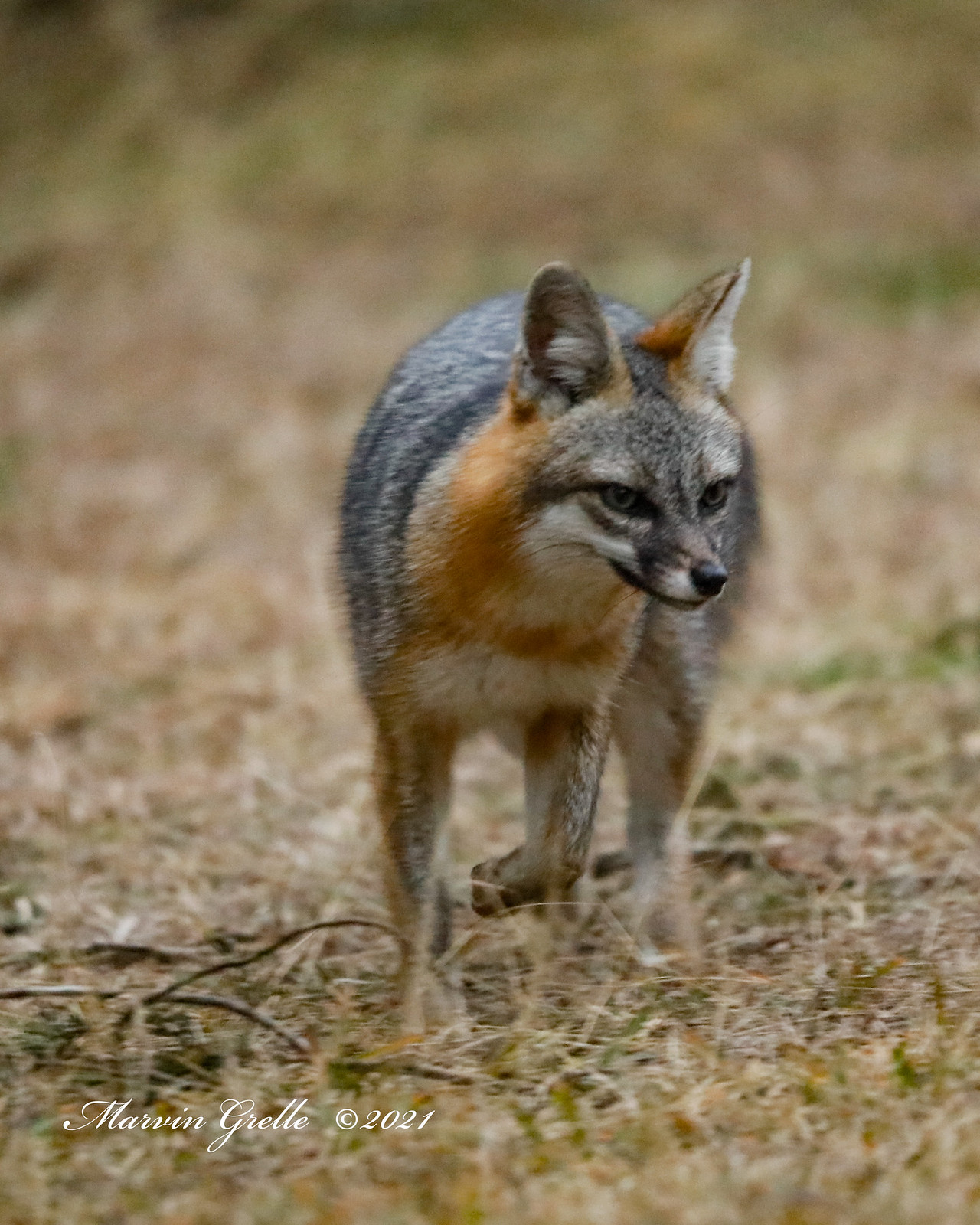This photo captures a wild animal reminiscent of a fox, set against a blurred backdrop indicative of an outdoor scene. The animal's coat exhibits a striking color contrast: a red and gold hue dominates its neck and chest, transitioning to a steel gray along its back and face, with touches of black and white near its slender snout that resembles a cat's face. The fox-like creature, roughly the size of a small dog, stands amidst a field of dry brush with scattered brown twigs and hints of green grass, all suggesting a late autumn or early winter setting. It gazes slightly to the right of the camera with both eyes open, one leg raised as if on alert while possibly hunting. Its ears stand erect atop its head, and a faint cream color traces down its neck. A visible watermark on the left reads, "Marvin Grell, copyright 2021," affirming the authenticity of the image.